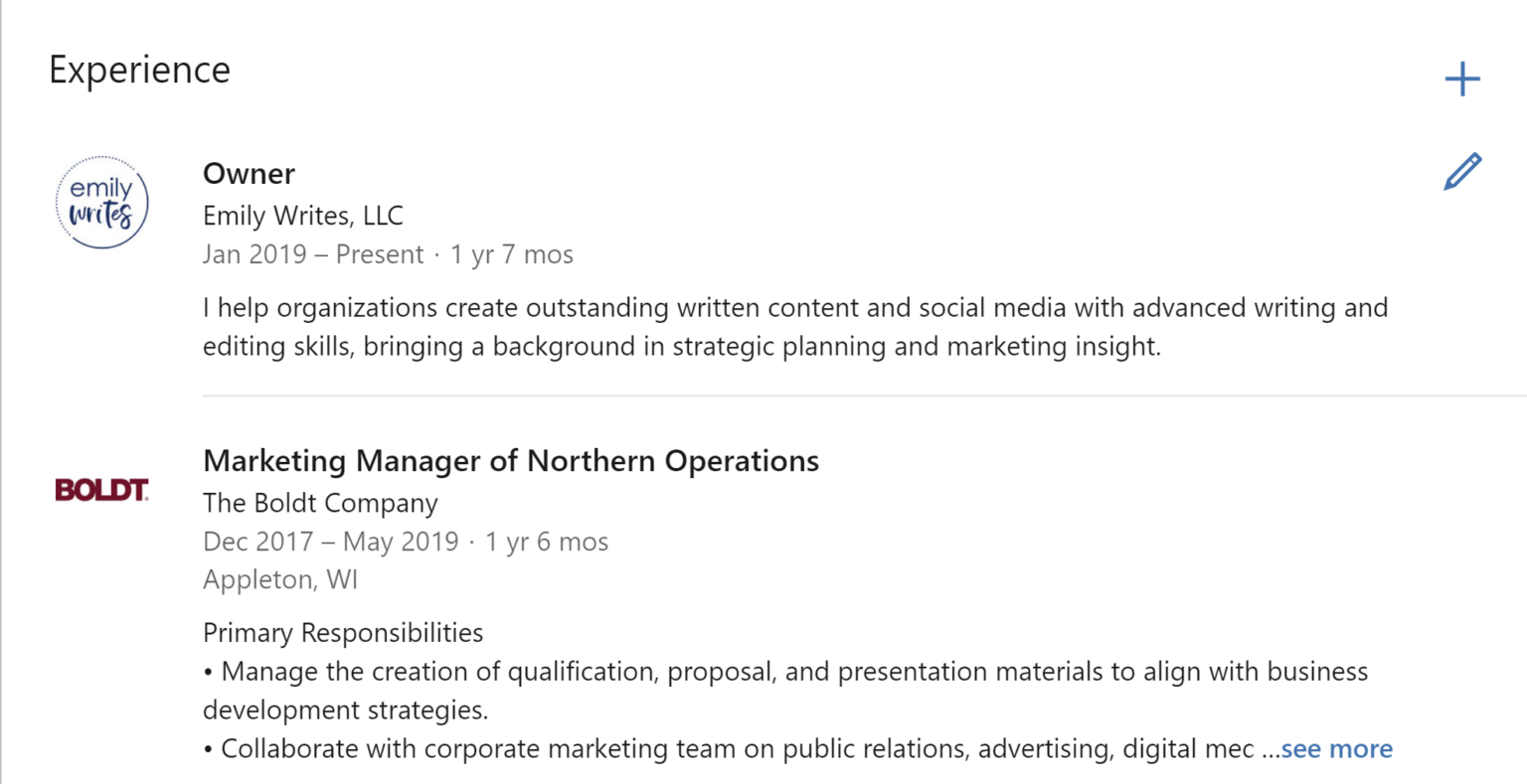In the top left corner, the word "Experience" is prominently displayed. Just below, there is a circle enclosing the name "Emily writes" in cursive, beside which the title "Owner" is written. Next to this, the company name "Emily writes LLC" is presented in uppercase letters, along with the employment duration: "January 19th - Present, 1 year 7 months." Below, a sentence elaborates, "I help organizations create outstanding written content and social media with advanced writing and editing skills, bringing a background in strategic planning and marketing insights."

A horizontal line separates this from the next section. To the left, the word "BOLDC" appears in a bold burgundy color. To the right, the title "Marketing Manager of Northern Operations, the BOLDC Company" is specified, with the employment duration: "December 17th - May 19th, 1 year 6 months." The location "Appleton WI" is mentioned, followed by the primary responsibilities:
 
• Manage the creation of qualification proposals and presentation materials to align with business development strategies.
• Collaborate with corporate marketing team on public relations, advertising, and digital MEC.

In blue text, an ellipsis followed by "See more" indicates additional information.